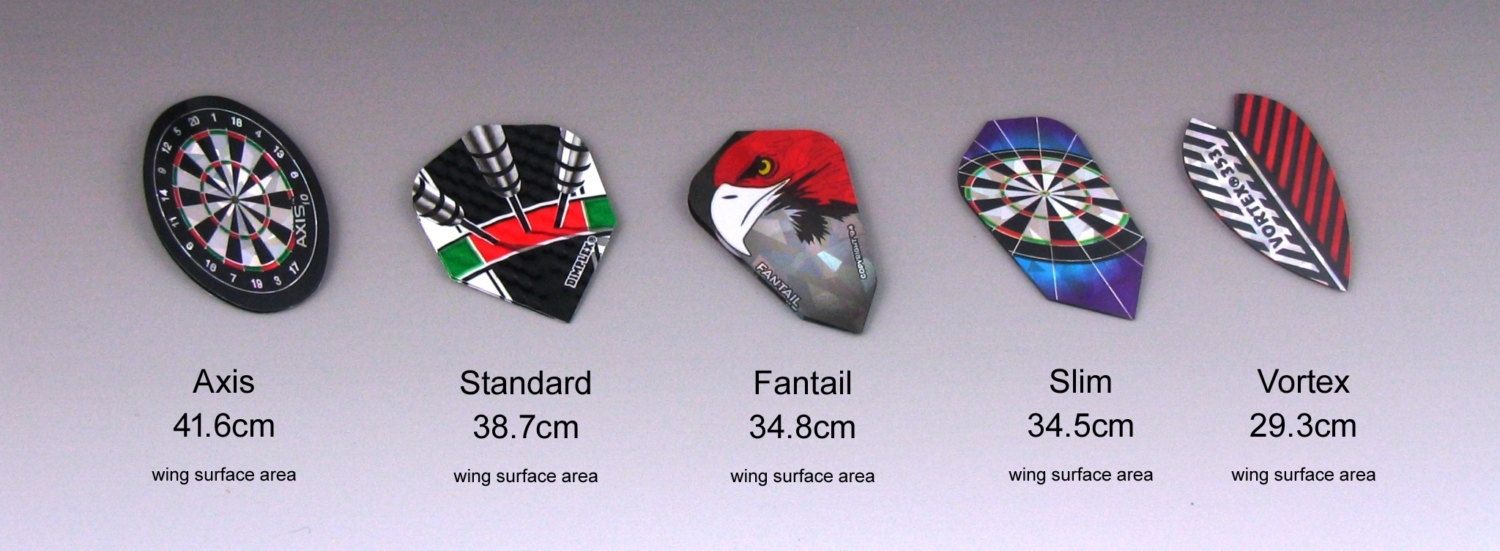This digital image serves as an advertisement for various dart-related items, prominently featuring five pictures arranged in a row against a grey background. On the leftmost side, there's an image of a dartboard labeled "Axis," with a wing surface area of 41.6 centimeters. To the right, a close-up of this dartboard reveals attached darts, illustrating "Standard," with a 38.7-centimeter wing surface area. The subsequent images show different types of dart tails with their respective sizes: "Fantail" (34.8 centimeters), "Slim" (34.5 centimeters), and "Vortex" (29.3 centimeters). These dart tails are depicted in various colors, including gray and red, blue, bullseye colors, and red with white and black stripes. The text below each image provides detailed specifications for each type, enhancing the advertisement's informative value.